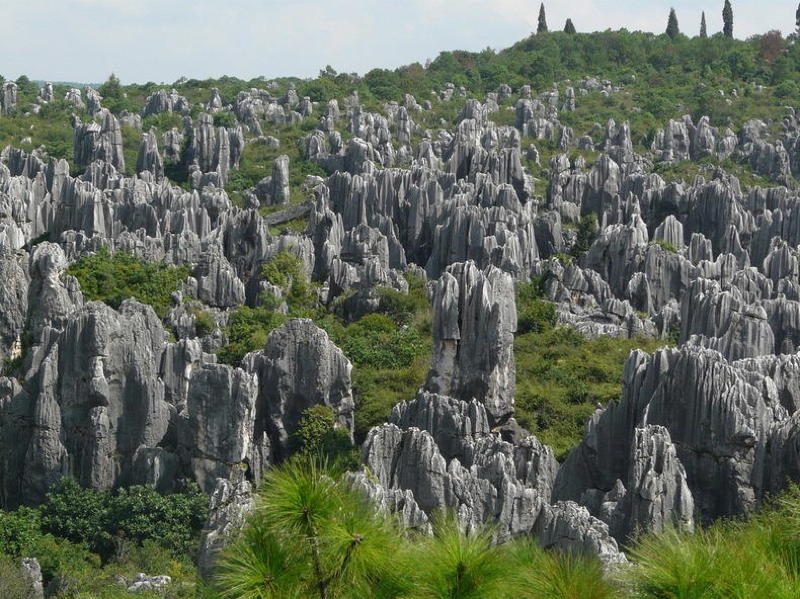This landscape photograph captures an expansive scene dominated by numerous jagged and sharply edged rock outcroppings, which appear to have erupted from the ground over time. The image is taken from an elevated perspective, possibly from a tree, as indicated by the pine needle branches visible in the foreground. The central subject consists of a striking array of rigid, gray rock formations, each varying in height and shape, giving a rugged, patterned appearance to the low hillside they inhabit. Interspersed among the rocks are patches of vivid green moss and clusters of bushes, adding a rich contrast to the grayscale stones. In the background, the gentle slope of the hillside rises to reveal the very tops of tall, slender conifer trees, reminiscent of Italian cypress, extending beyond the crest. The overall color palette of the photograph is a harmonious blend of varying shades of green from the plant life and grays from the rocks, with subtle hints of white on the stones, showcasing the natural beauty of erosion and growth in this serene, untouched landscape.